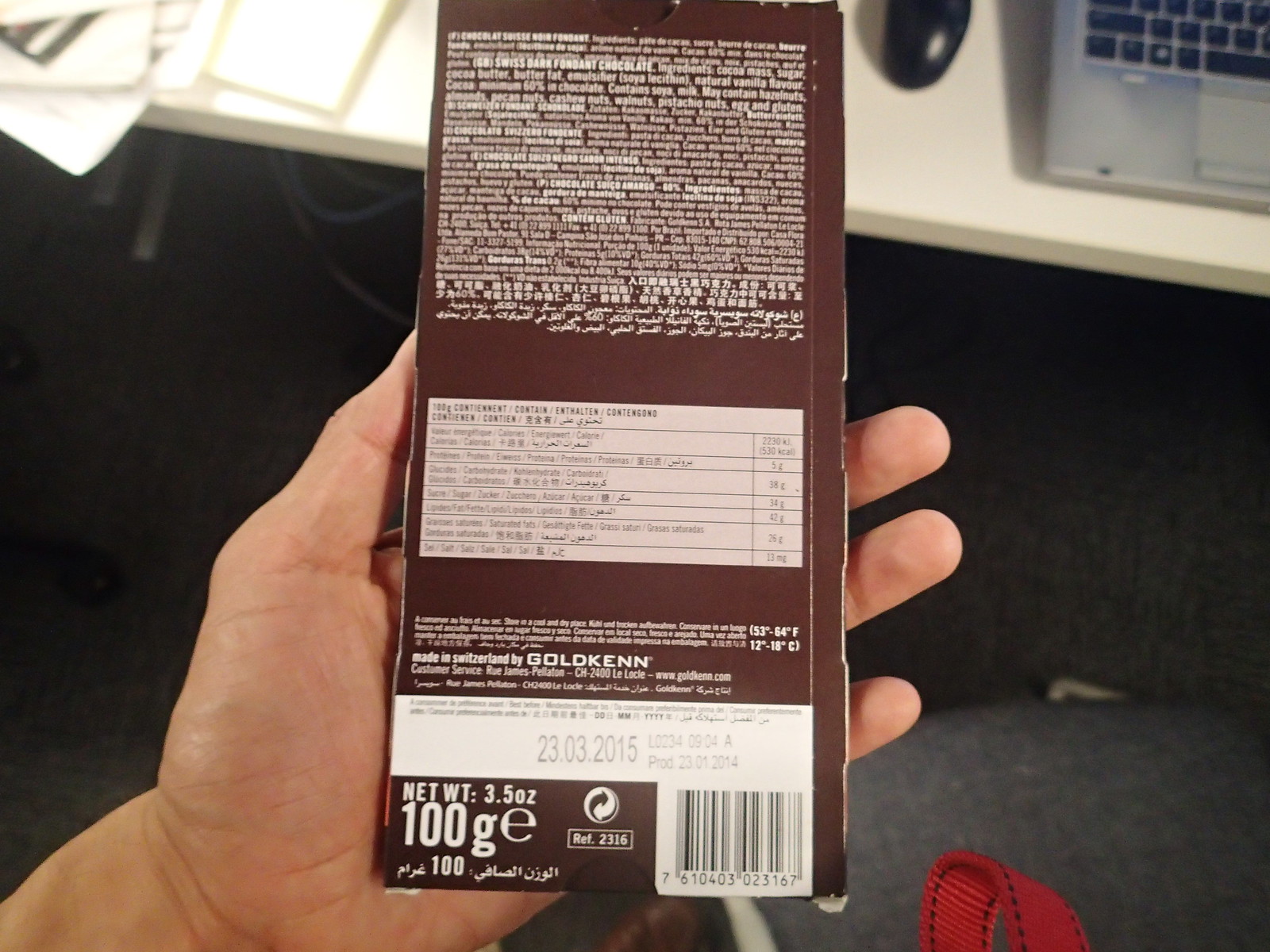In this horizontal rectangular photograph, a light-skinned hand emerges from the bottom right side into the center, holding a chocolate brown candy bar wrapper with nutritional information in an unreadable, small white font. At the top of the wrapper is bold, white text, and in the middle is a white rectangular box containing more writing, including the text "Net weight: 3.5 OZ" and "100G." The barcode appears in the bottom right corner of the wrapper. The person is seated at a white desk cluttered with cords and white papers on the left, and uses a silver laptop with black keys and a black mouse. A faint shadow is cast by the keyboard. The floor features Berber carpeting and a blue office chair, and to the right is a red bag handle. The photograph is well-lit from the left, highlighting the detailed workspace.